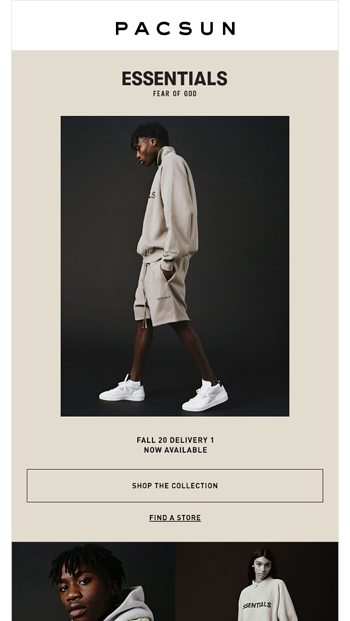In this clothing advertisement from PacSun, the brand's name is prominently displayed at the top. Just below "PacSun" is the sub-heading "Essentials," followed by "Fear of God." The central image features a man walking to the left, dressed in a gray sweater, gray shorts, and white shoes. The entire scene is set against a black background. Beneath the picture is the caption "Fall 20, Deliver 1, Now Available," followed by a prominent rectangular button labeled "Shop the Collection." Further down, there's a link to "Find a Store." At the bottom of the advertisement, there are partial, cut-off images of a man and a woman, suggesting additional clothing options.